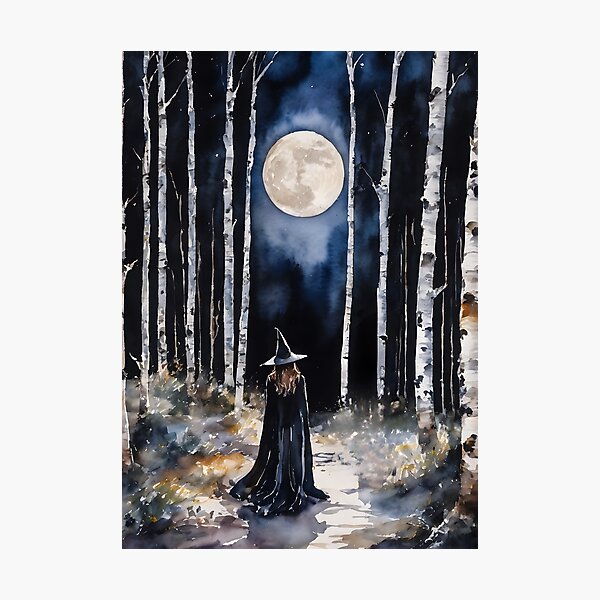The image is a delicate watercolor painting depicting a young witch walking through the woods at night. She stands in a moonlit clearing, facing a prominent, luminous full moon in a night sky that transitions from black to blue. The witch, seen from the back, wears a pointy black hat and a long black cape that drapes to the ground. Her brown hair cascades down her back. She is walking on a light-colored path surrounded by varying shades of white, brown, and beige grass, with some bushes nearby. Slender white birch trees and thin branches frame the scene on both sides, their white bark contrasting starkly with the dark sky. The moonlight bathes the landscape, creating a mystical atmosphere and casting a shadow of the witch.